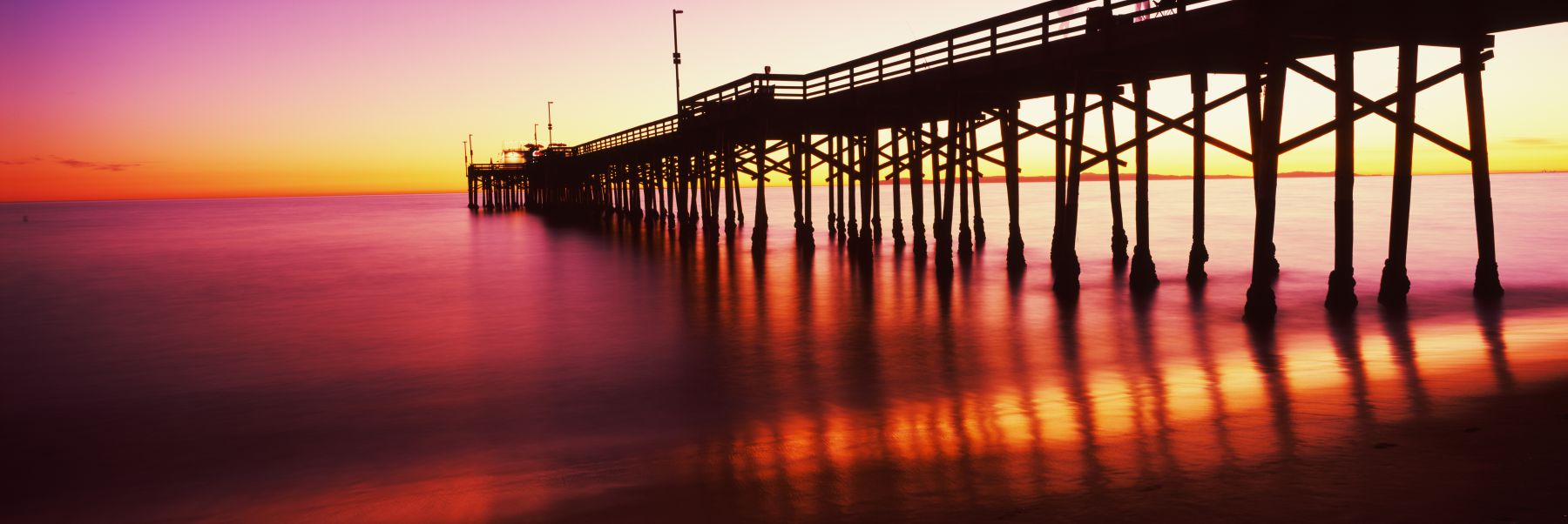This stunning photograph captures the serene beauty of a long pier stretching into a calm body of water, likely an ocean or inlet, during an enchanting sunset. The sky is painted in vibrant hues of purple, pink, and orange, creating a mesmerizing gradient that transitions from brighter shades near the shore to deeper tones higher above. The still water mirrors this colorful sky almost perfectly, adding to the tranquil ambiance with its glass-like surface that reflects the purple and other warm shades. The silhouette of the pier, with its visible fence, streetlights not yet illuminated, and multiple supports descending into the water, adds a striking contrast to the colorful backdrop. There are no people, boats, or activity, highlighting the peacefulness of the scene. The horizon glows with the beautiful colors of dusk, making it a picturesque and quiet evening by the water.